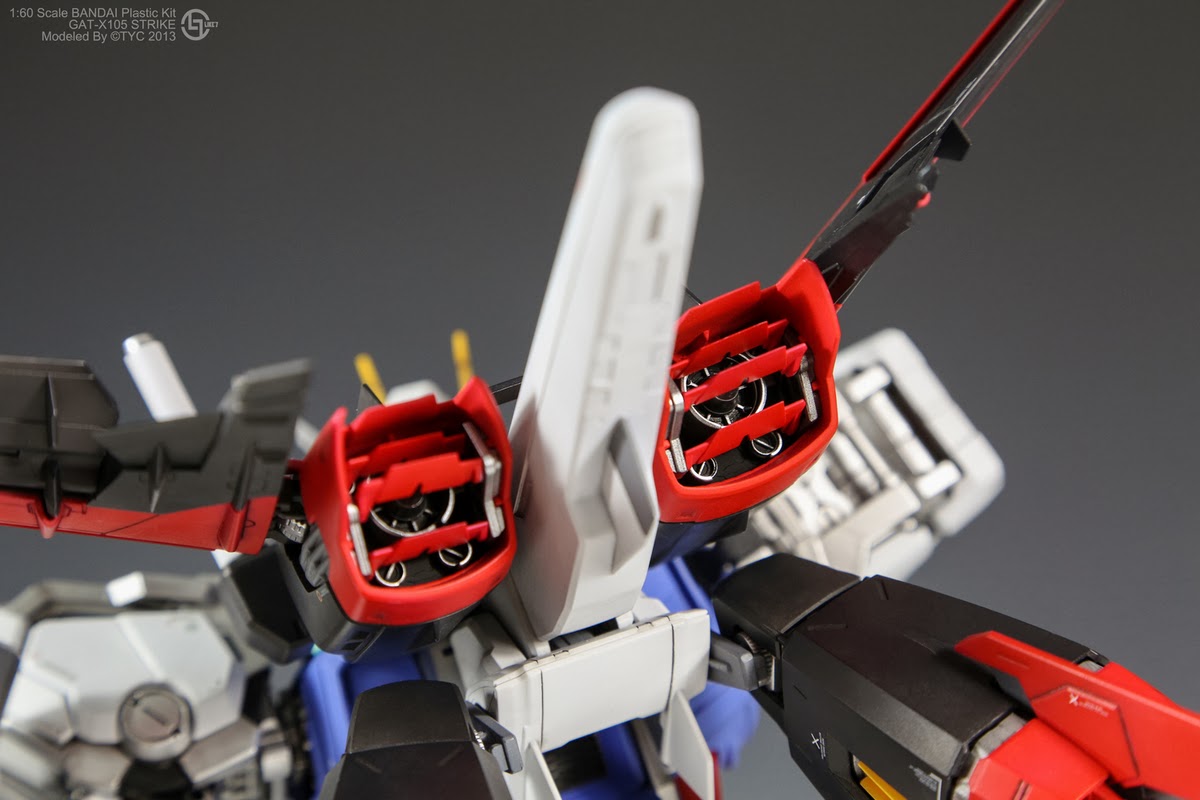The image showcases a close-up of a complex, detailed model of a transformer or robotic toy, specifically a 1/60th scale Bandai plastic kit identified as GAT-X105 Strike, modeled by TYC in 2013. The photograph provides an intricate view of what appears to be the underside of the transformer, highlighting a variety of shapes and components in colors like black, red, white, silver, and gray. Noteworthy features include pointed angles and gears visible through transparent parts, which are interestingly attached using silver metal arms and plastic screws. The model includes distinctive elements such as red-marked black engines, a white tailpiece, and wings, all suggestive of a plane-like transformation. The backdrop is a grey background with text indicating the model's specifics, providing a clear view of the technical and aesthetic complexity of this transformer model.